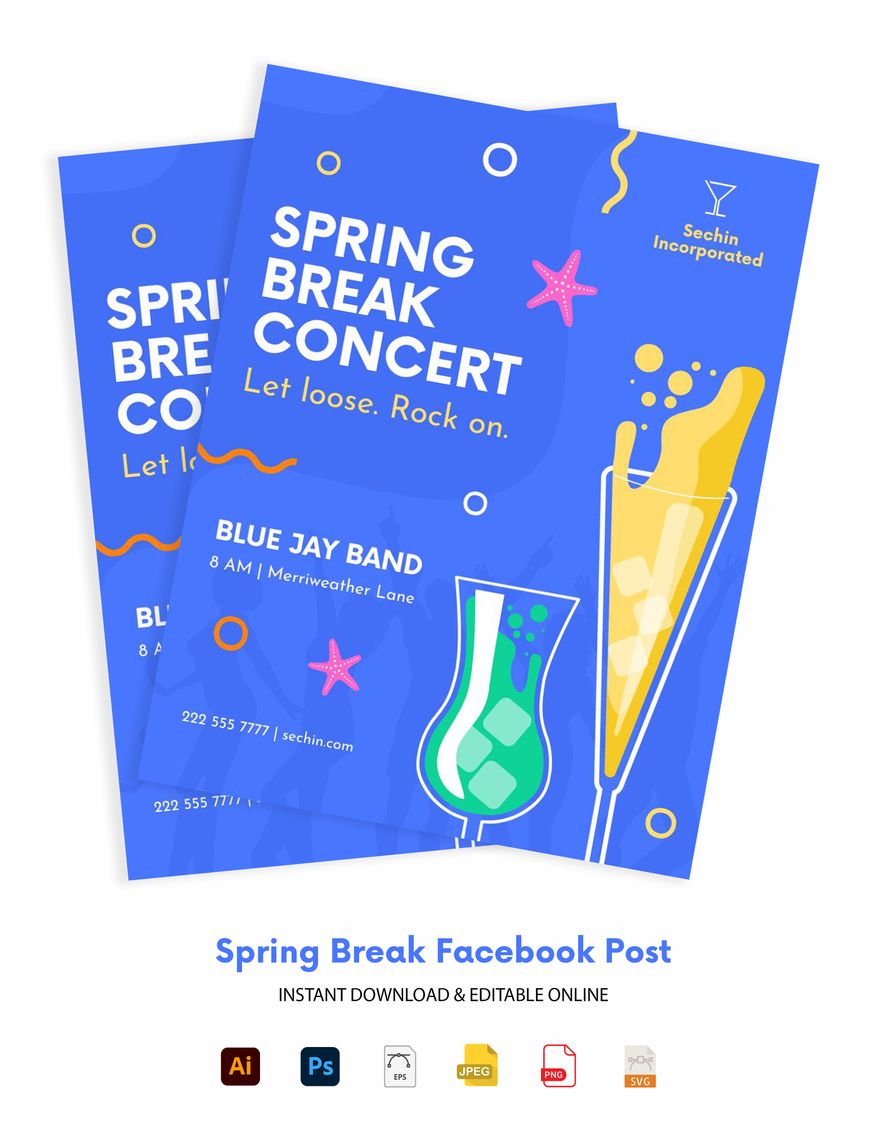This image features a computer graphic of a Spring Break Facebook post, prominently showcasing a blue card with detailed event information. The card, angled and overlaid on an identical one, reads "SE Sechin Incorporated" in white text at the top, followed by "Spring Break Concert, Let Loose, Rock On" in gold letters. It advertises a performance by the "Blue Jay Band" scheduled for 8am at "Merriweather Lane," with a contact number "222-555-7777" and the website "sechin.com." To the right, there are graphics of two dainty glasses; one is a shorter glass with green liquid, and the other is a taller martini glass with yellow liquid. The background includes pink stars, a squiggle on top, and small icons for instant download file formats such as AI, PS, EPS, JPEG, PNG, and SVG. The overall design has a playful layout with elements like a yellow squiggle and pink starfish, making it visually dynamic on a white background.